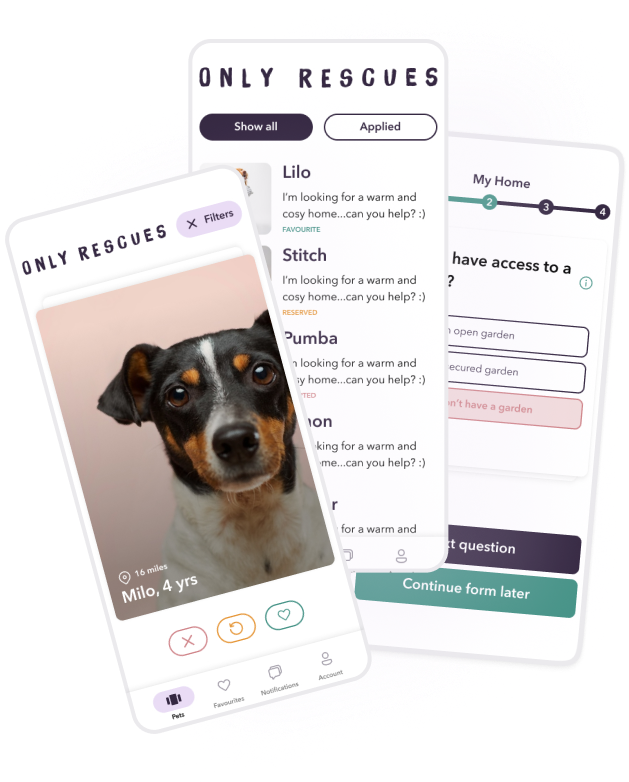The image depicts three simulated phone screens displayed against a white background, arranged like a fanned-out hand of cards.

1. **Left Screen:**
   - Positioned at a slightly steeper than 45-degree angle up to the right.
   - Header with "ONLY RESCUES" in all capital letters on a white background.
   - To the right of the header, there's a purple button with a black 'X' icon, followed by black text that says "FILTERS."
   - Below the header, there is a vertical photograph of a dog against a pink backdrop. The dog has a black and brown face with a white stripe down its front and the left side of its snout, and a predominantly white body with some brown spots.
   - Overlapping the bottom left of the photo, there is a dark gradient with white text that reads "MILO, four years."
   - A white geolocation pin icon is located next to text indicating "16 miles" in small letters.
   - At the bottom of this screen, there are three pill-shaped icons with white backgrounds and colored outlines: a red 'X', an orange refresh symbol, and a green heart.

2. **Middle Screen:**
   - Appears more vertical.
   - Features a header similar to the left screen with "ONLY RESCUES" in all capital letters on a white background.
   - Beneath the header, there are two buttons with rounded edges: a purple button on the left with white text that says "SHOW ALL" and a white button with a purple outline and text that says "APPLIED."
   - A list of animals begins below the buttons, but the content is partially obstructed by the overlaying left screen. Visible text includes "Lilo," followed by "I'm looking for a warm and cozy home. Can you help?" with a smiley face emoji.
   - The word "FAVORITE" appears beneath this in green text.

This detailed arrangement showcases an application interface focused on adopting rescue animals, with features such as filtering options, an animal profile with location and interaction buttons, and a list of potential pets.